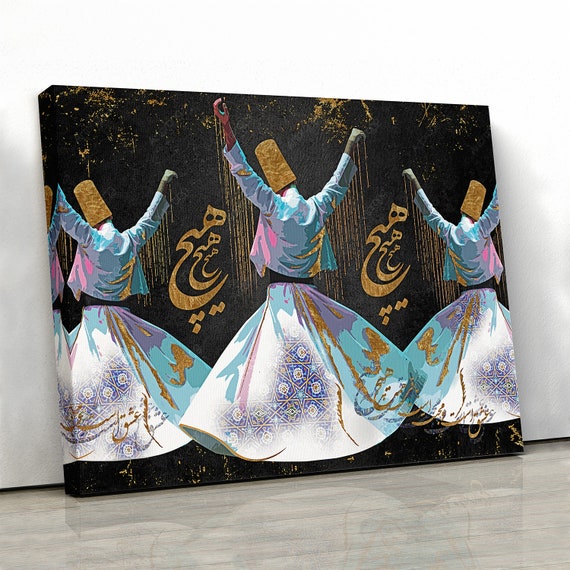The image depicts an expressive indoor artwork, possibly a painting, leaning against a white wall and resting on a taupe wooden or marble-like floor. It features three individuals, likely members of an Indian tribe, poised in a dynamic dance pose with their hands extended upwards to form a Y shape. 

The figures are dressed in cultural attire that includes long, flowy skirts and matching tops adorned with intricate designs, primarily in purple, blue, white, and gold. The skirts appear to be ballooned out, suggesting a spinning motion. Their attire also features astrological symbols and crescent moons, which are echoed in the golden patterns both on the background and on their clothing. Each dancer wears a tall, thin cylindrical gold hat.

The background of the canvas is a rich mixture of black, yellow, and green, with what appear to be abstract representations of trees. Notably, the individuals are shown from the back, emphasizing the ornate detailing of their attire. The entire artwork is framed with gold accents, adding a sense of depth and luminance to the piece. This detailed and vibrant painting could likely be found in an art gallery or as a stock image on a website.